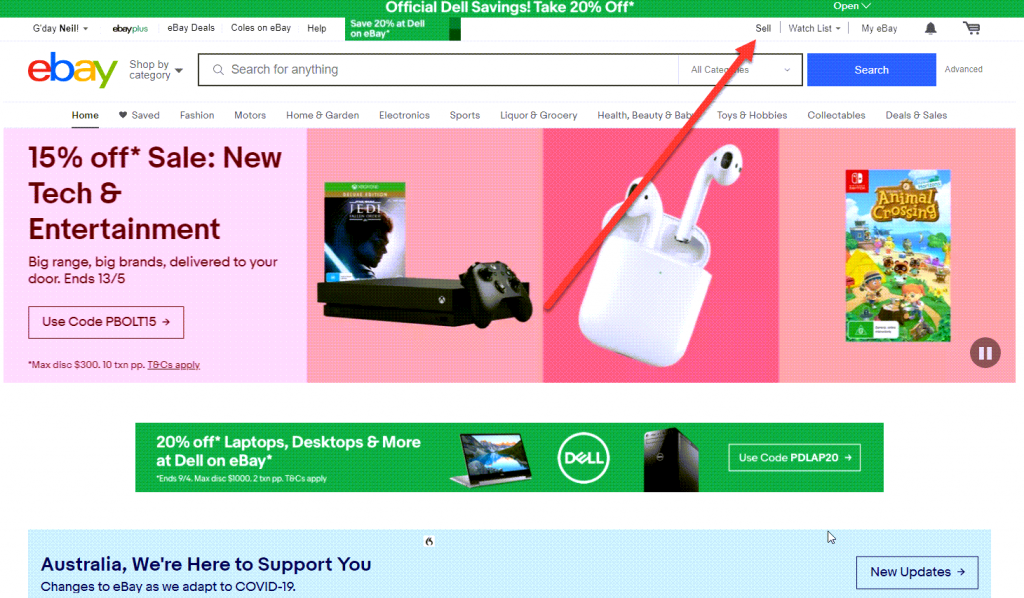This image captures a screenshot of the eBay website homepage. Dominating the upper left corner, the iconic eBay logo is prominently displayed with the letters 'e' in red, 'b' in blue, 'a' in yellow, and 'y' in green. 

Stretching across the top of the page, a noticeable banner declares "Official Dell Savings: Take 20% off*" in the middle. Adjacent to this announcement on the right side, there is an interactive dropdown menu labeled "Open" accompanied by a down arrow.

Central to the page is a vibrant advertisement boasting a 15% discount on new tech and entertainment products. The promotional text promises a wide range of big brands delivered right to your door with a specified date, 13/5 (May 13th), and instructs users to apply the code "PBOLT15" to avail the offer. An asterisk notes a maximum discount of $300.

In this promotional area, several product images are displayed: 
1. A copy of the Xbox game "Jedi Survivor."
2. An image, seemingly of the Xbox One console.
3. A red error icon adjacent to a symbol designating a sale.

Additionally, a pink section highlights a pair of AirPods, while another dark pink square on the right showcases a set of items including the box for the Animal Crossing edition of the Nintendo Switch. The layout of this advertisement is visually segmented, each section drawing attention to various tech and entertainment deals available on eBay.